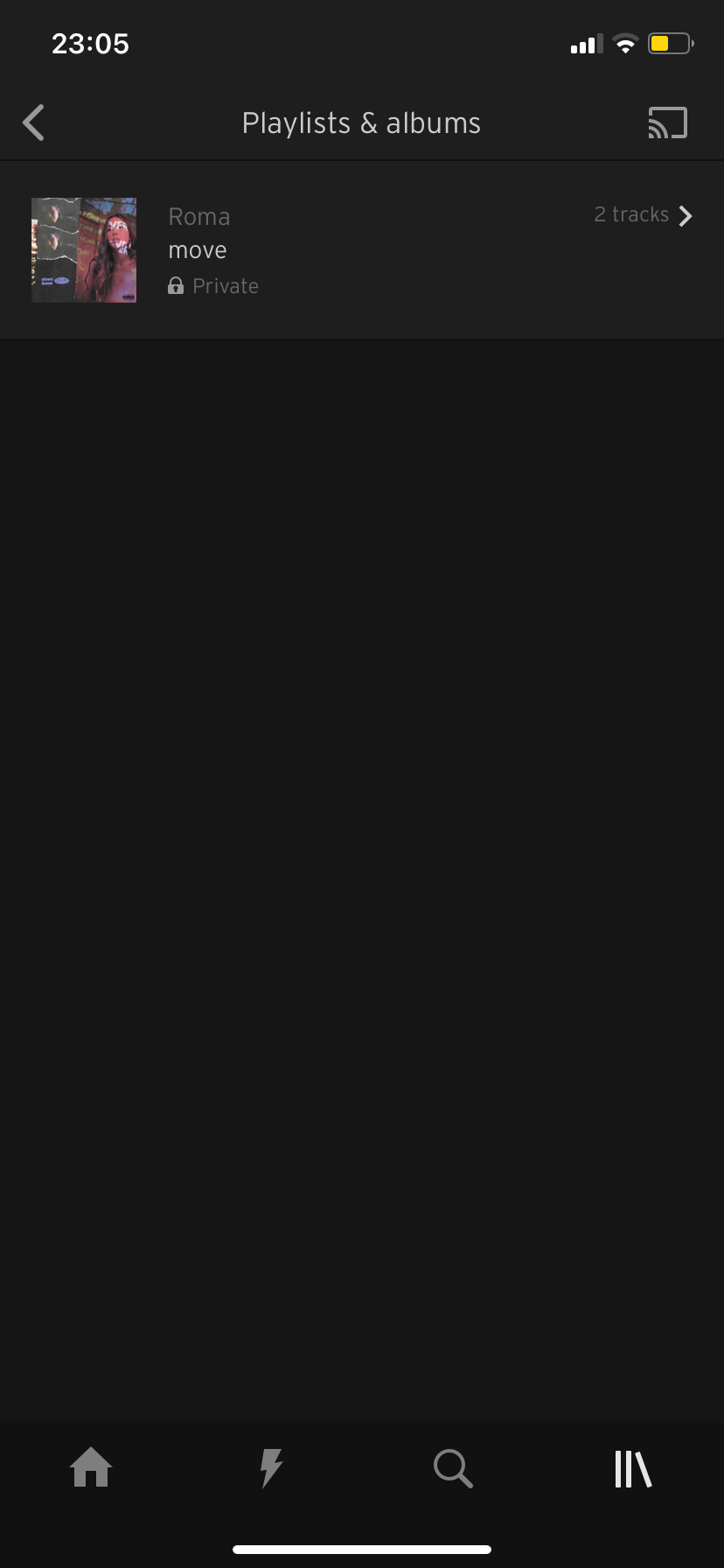This detailed caption captures the essence of the screenshot:

"This screenshot, likely taken on an iPhone, displays various interface elements indicating time, connectivity, and app features. The time in the top-left corner reads 23:05. Cellular and Wi-Fi connections are active, and the battery level is around 40%, with the device in Low Power Mode. The top section of the screen shows tabs labeled 'Playlists' and 'Albums,' with the 'Playlists' tab currently selected. It displays a single playlist named 'Roma,' containing two tracks and marked as private. The playlist features two track icons. At the bottom of the screen, there are four navigation icons: a home symbol, a lightning bolt, a magnifying glass for search, and an icon with two vertical lines and one diagonal line, which appears to be selected, possibly indicating the current view mode for Playlists and Albums. The background is black, suggesting that the device is in dark mode."